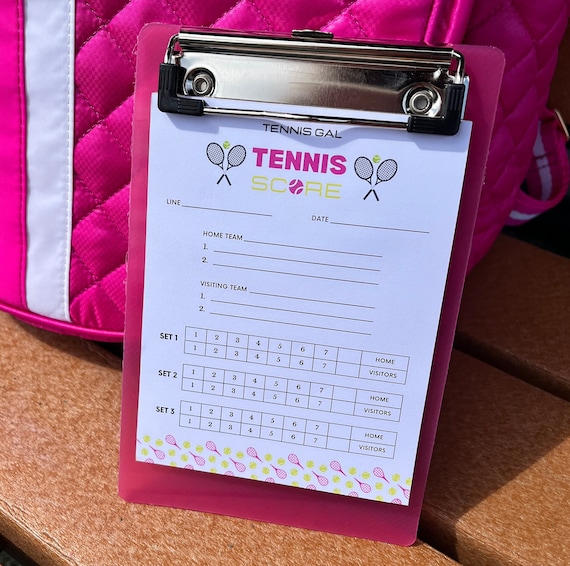The photograph captures a pink clipboard with a chrome top that holds a piece of paper titled "Tennis Gal Tennis Score." The paper features spaces to input details such as the date, home team, visiting team, and outlines three sets for scoring each game. The layout includes lines labeled Line, Date, Home Team, Visiting Team, and numbered sections 1 to 7 for both teams. Additional illustrations of crossed tennis rackets flank the title and are also printed at the bottom of the page in pinks and yellows. The clipboard is situated on a wooden, slatted brown bench, with a pink gym bag featuring a white stripe down both the middle and the handles resting behind it.